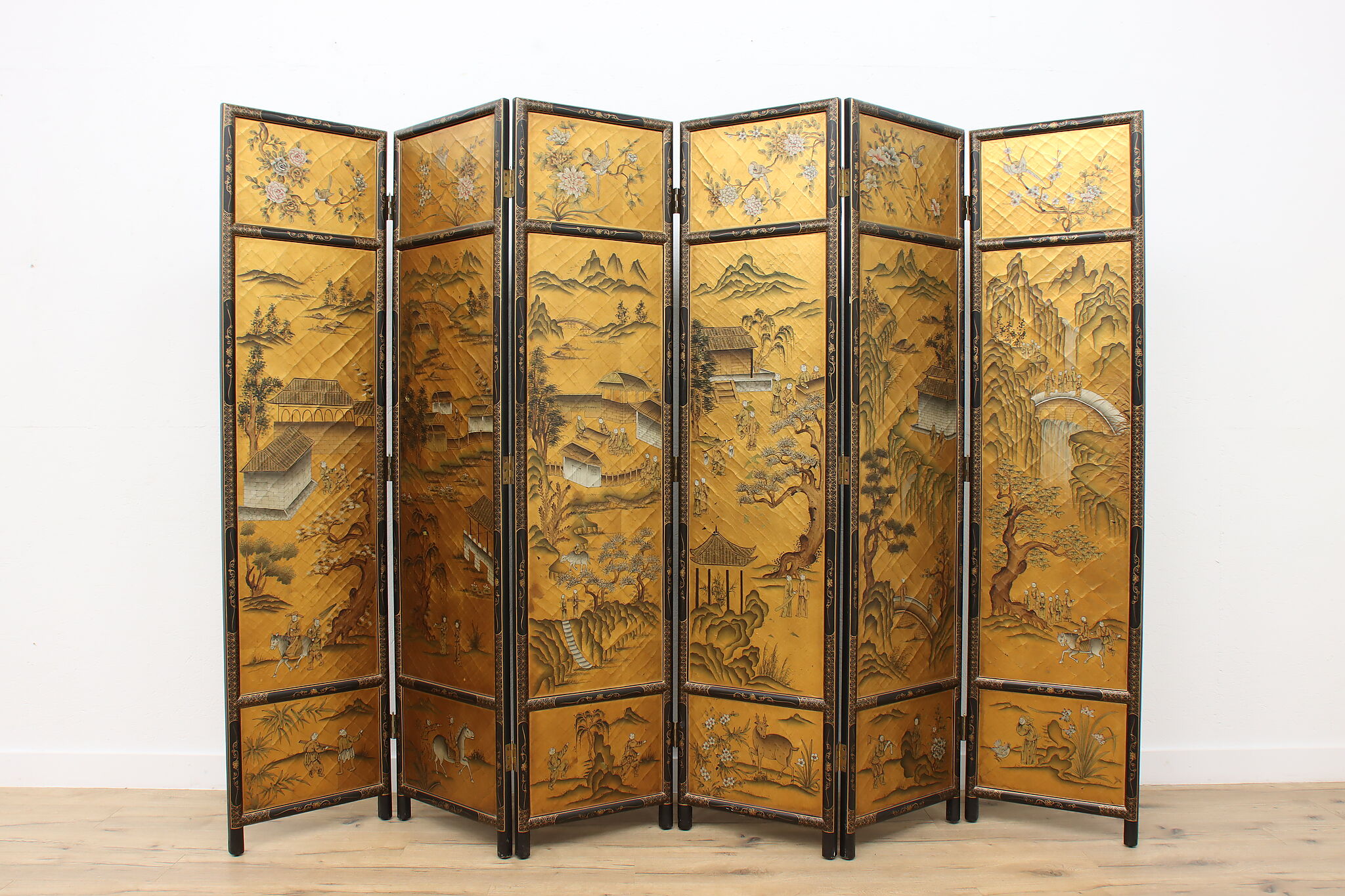This image captures a detailed Japanese folding screen, characterized by its intricate artistry and refined presentation. The screen, composed of six tall, foldable panels with a rich brownish-gold trim, stands against a backdrop of white walls and a light wooden floor. Each panel is adorned with a complex, gold-painted design featuring muted greens, whites, and browns to illustrate varied scenes. 

On the far right, a mountainous landscape is depicted with a bridge and trees below it. Moving leftward, another mountain scene unveils a building perched on its incline with more bridges, distant mountains, and clusters of trees. The central segments reveal a bustling village with people and trees interspersed throughout, transitioning to a lively ravine area where steps lead down into it, accompanied by more buildings and distant mountains.

The far-left panels present a close-up view of ornate buildings, further accentuating the screen’s exquisite detail. Along the bottom portion of these panels, various animals are intricately painted, while the top showcases delicate depictions of flowers. The screen stands slightly elevated on small feet, giving it an accordion-like structure that can be easily folded flat if needed. This ornate and visually rich screen serves as both a functional room divider and a piece of art, encapsulating the beauty and traditional artistry of an oriental village.